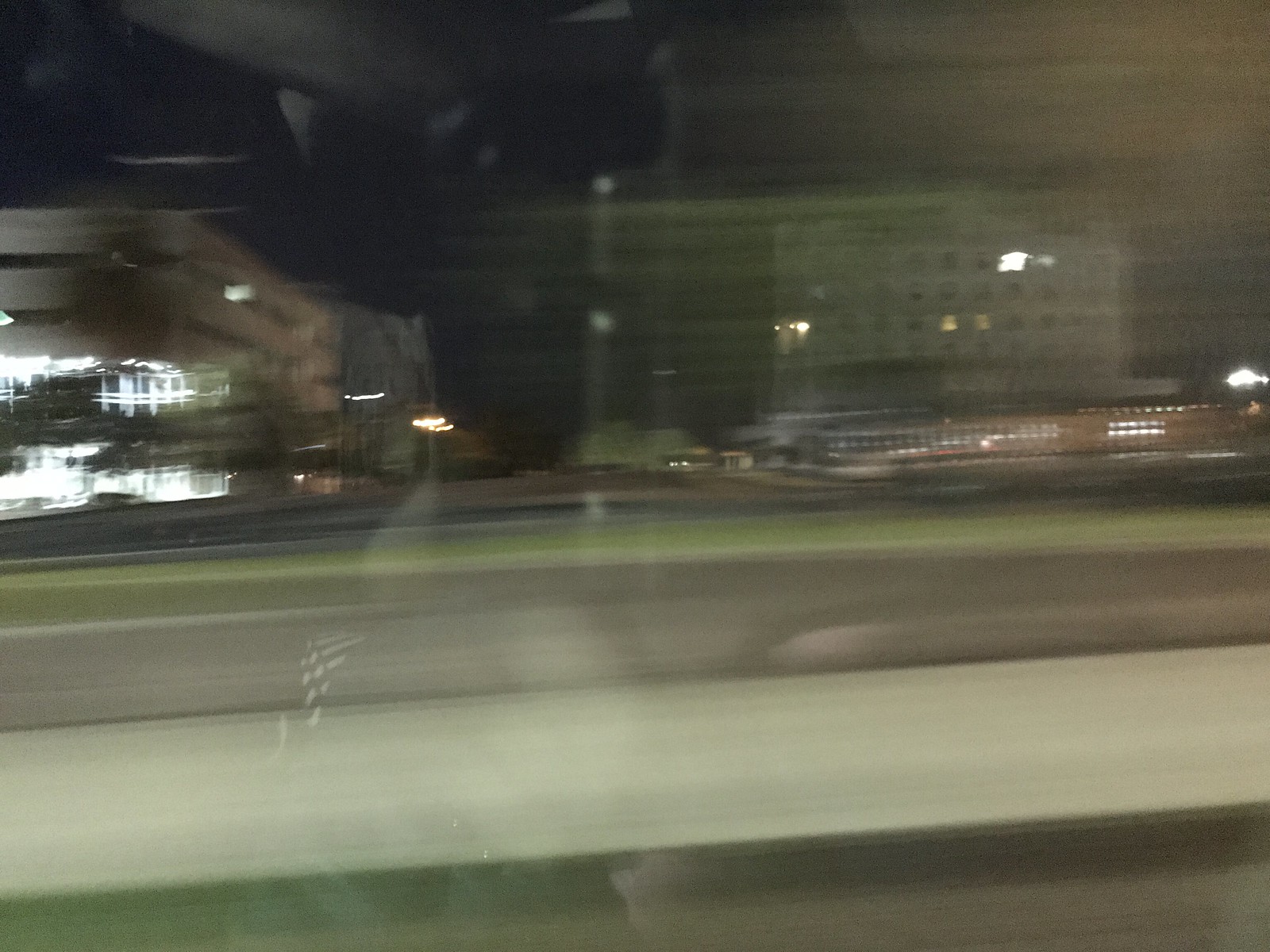A blurry nighttime photograph taken from the inside of a moving vehicle, possibly a bus or a car, obscures many of its finer details. The image depicts a road flanked by buildings on both sides: a large, gray, industrial structure or hospital on the right, and a lower building that might be a parking garage on the left, identifiable by openings on its upper levels and brightly lit lower floors. The dark road is divided by a guardrail or lane divider, beneath which lies a patch of green shoulder. Reflections off the vehicle's window, such as a white rim, add to the image's overall lack of focus, alongside possible moisture streaks on the bottom center. The night sky looms pitch-black above, with only a few random lights visible in the skyscraper's windows and various reflected areas from inside the vehicle.